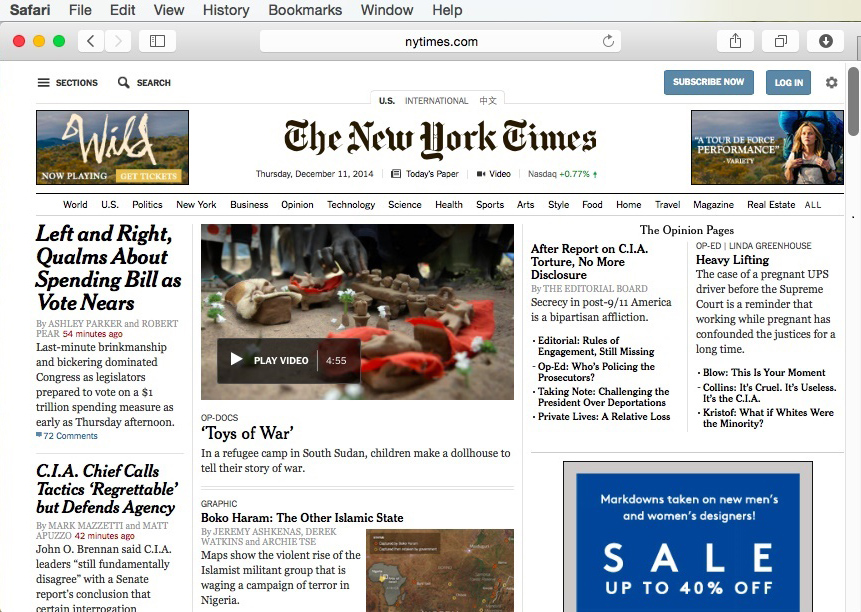**Screenshot from the New York Times Website - December 11th, 2014 Edition**

This detailed screenshot from the New York Times website, dated December 11th, 2014, prominently features the following highlights:

1. **Main Headline**: "Wild and Outplaying: Tour, Divorce, Performance, Variety"
   - **Featured Actress**: Reese Witherspoon
   - **Focus**: A movie involving Reese Witherspoon, discussing her tour, divorce, performance, and variety.

2. **Articles Summary**:
   - The section includes a list of seven articles displaying a mix of themes such as love, joy, and other prompts, contributing to a diverse range of topics for readers.

3. **Video Feature**:
   - **Title**: "Toys of War in Rooftop Camp in South Sudan"
   - **Description**: Children in a South Sudan camp build dollhouses to narrate their experiences of war.

4. **Promotional Content**: 
   - There is a notable sale announcement of 40% off, highlighted in blue, attracting readers’ attention.

5. **Other Noteworthy Articles**:
   - **Boko Haram**: Coverage on the militant group Boko Haram, exploring a perspective titled "The Other Side."
   - **Law-Enslaving State**: An article addressing the concept of a "Law-Enslaving State."
   - **CIA Chief**: A piece on the CIA Chief defending the agency amid active regrettable circumstances.

This screenshot encapsulates the diverse and engaging content offered by the New York Times on this particular date, highlighting significant news stories, human interest pieces, and promotional offers.